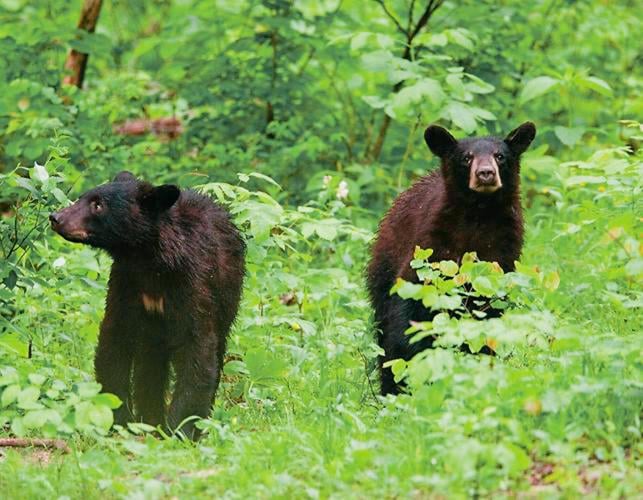In this photograph, taken in a lush, green forest, two juvenile bears, likely grizzly or black bear cubs, are depicted amidst dense foliage. The vibrant greenery includes an array of tall grasses, shrubs, and tree trunks. Both bears are dark brown but exhibit variations in their fur coloration. The bear on the right, slightly larger, has a brown coat with black furred legs and lighter brown markings around its snout and nose. Its ears are perked up, and it looks directly into the camera with an alert expression. The bear on the left, appearing somewhat smaller and perhaps more timid, has shorter ears and is gazing off to its left. It features a similar dark brown and black fur combination, with noticeable lighter patches on its muzzle and chest. The rich details of their surroundings, with trees and foliage almost reaching the bears' height, enhance the image's depth, capturing a serene yet captivating moment in the wild.